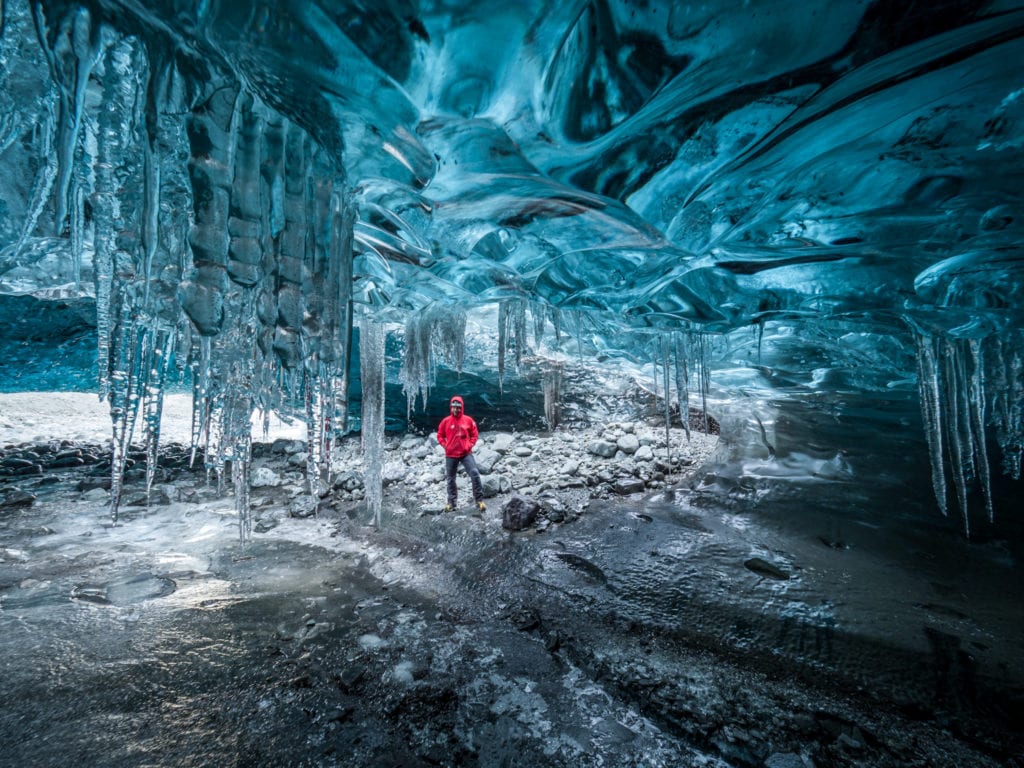This full-color photograph, taken outdoors during the daytime in an extremely cold environment, captures the captivating scenery of an ice cave. The square image features a small, distant figure standing in the center—a person dressed in a red hooded jacket, likely a man, with dark gray pants and tan boots. His hands are tucked into the front pockets of his hooded sweatshirt, and he appears to be wearing a hat underneath the hood. The cave's ceiling is made of stunning blue ice, almost glowing, adorned with intricate and extensive icicles that hang down in various directions and lengths, some forming vertical lines ending in sharp points. The ground beneath him is a dark, blackish-gray surface, with some large, light gray rocks visible behind him. The primary focus is the mesmerizing ceiling of the cave, with its beautiful ice formations creating a surreal, almost otherworldly atmosphere.